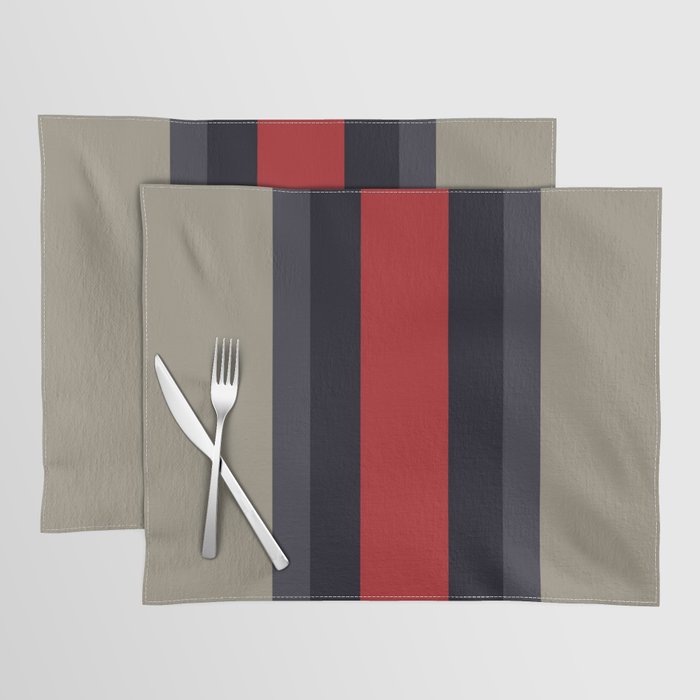This professional studio photograph captures two rectangular dining room placemats with a symmetrical design, placed on a light gray background. The top placemat is positioned centrally with a polished silver fork and knife arranged diagonally on the lower left. Each placemat features a series of horizontal stripes: a bold red stripe in the center, flanked by black stripes, then thinner dark gray stripes, and finally, outermost stripes in a grayish green-beige color. The identical placemat beneath is partially visible. The precise white stitching along the edges and the polished cutlery suggest a high-end dining setup, enhanced by the excellent studio lighting that highlights the textures and colors.